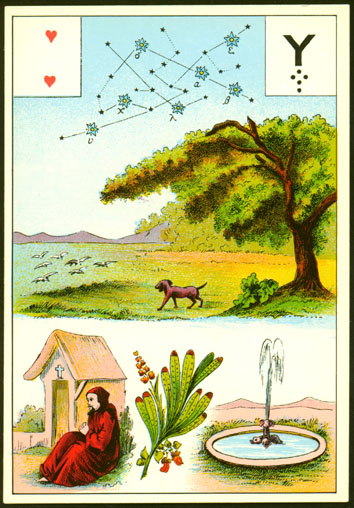This meticulously detailed drawing is divided into two distinct halves, each richly illustrated with vibrant scenery and intriguing symbols. 

The top half features a serene prairie bathed in daylight, with a striking blue sky adorned with clearly visible constellations. At the center of the prairie stands a majestic dog, surrounded by lush green grass. On the right side of the scene, a towering tree provides a sense of scale and tranquility. To the dog's left, a group of ducks contributes to the natural ambiance. In the distant background, the outlines of mountains complete this idyllic landscape. Two hearts are vertically aligned in the top left corner, while the top right corner showcases the letter 'Y' accompanied by five dots arranged in an upward-pointing arrow formation just below it.

The bottom half of the drawing shifts to a more tranquil, spiritual scene. A monk is seated on the left side next to a modest chapel made of straw, which features a narrow door almost as tall as the sitting monk and a small engraved blue cross. To the right of the monk, a large leaf from a nearby plant adds a touch of nature to the scene, complemented by a fountain that shoots water upwards. This section also presents a clear blue sky and distant mountains, tying both halves together with a consistent natural theme.